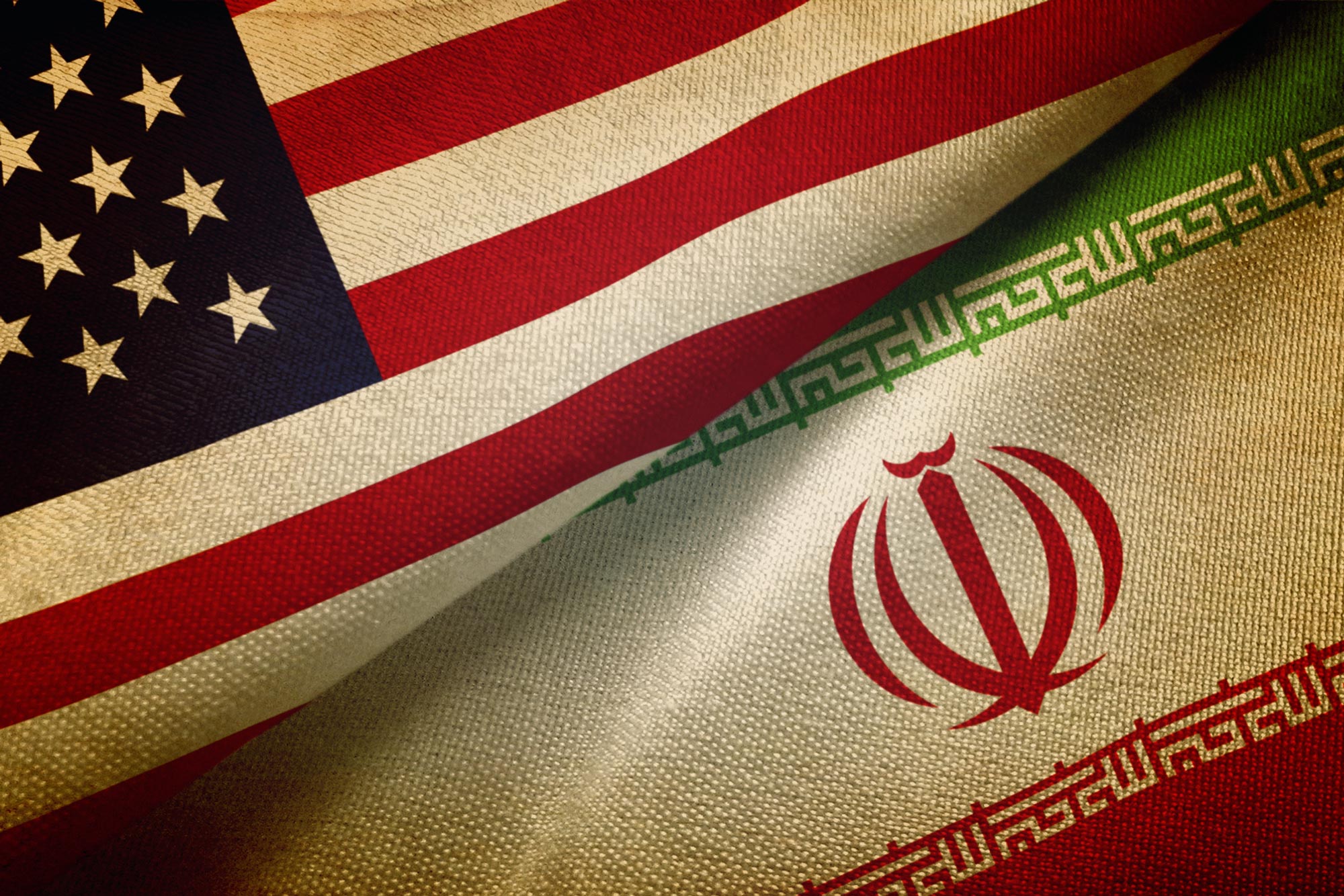This close-up color photograph captures two overlapping fabric pieces printed with national flags. The top fabric prominently features the American flag, exhibiting several white stars on a blue field in the upper left corner, along with visible red and white stripes, although some stripes are folded and partially obscured. Beneath it lies the Iranian flag, characterized by a green stripe at the top, a white middle section adorned with a red decorative emblem and intricate border designs, and a red stripe at the bottom. The flags are neatly arranged, providing a striking contrast between their distinct national symbols and colors.